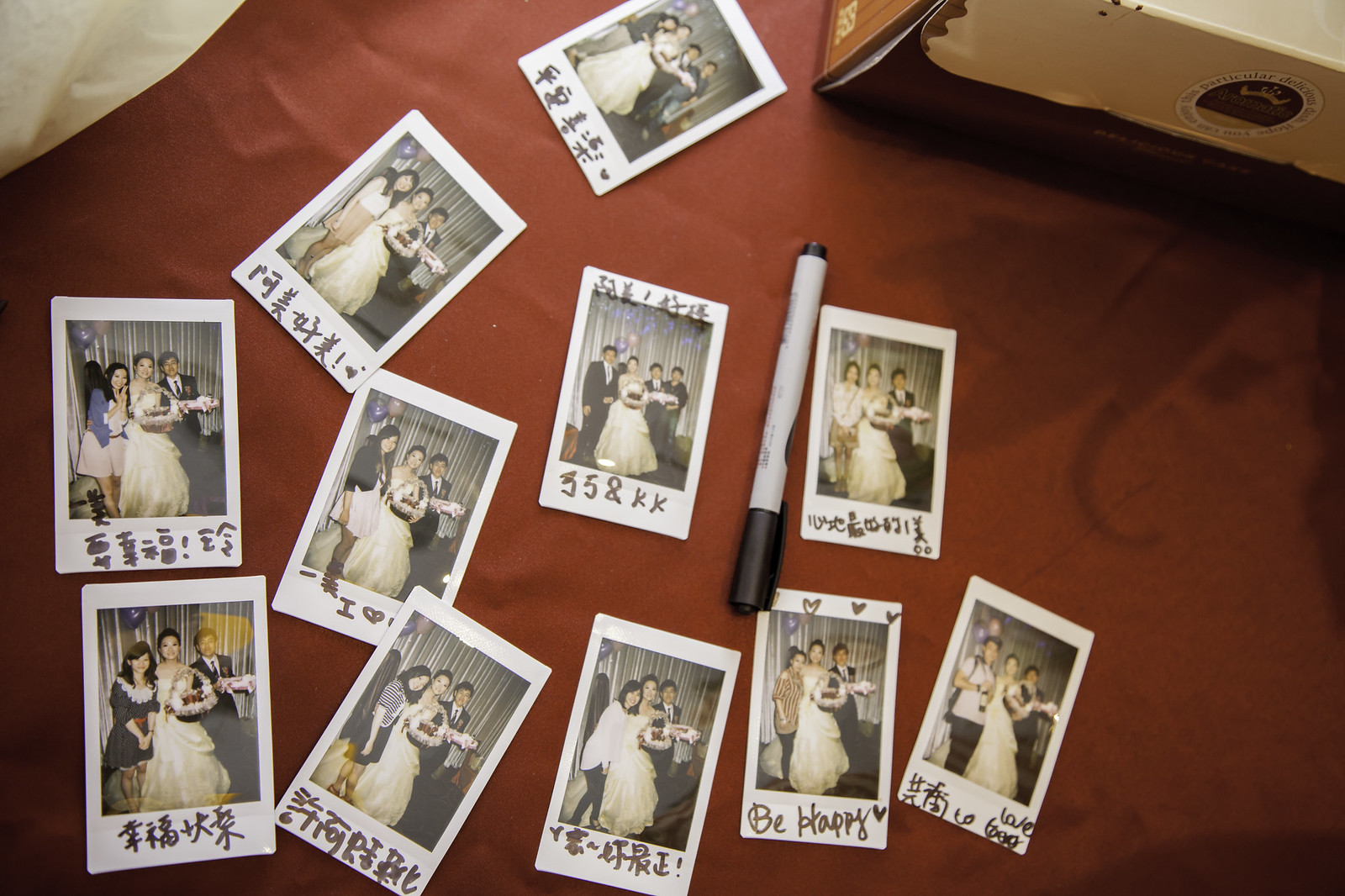This image is an overhead shot of several Polaroid wedding photographs spread out on a red tablecloth or blanket. In the background, on the top right, there is a brown shoebox with a light brown lid. The photographs are arranged in a pattern, with most of them featuring the bride in her long white dress posing with family and friends. The top row has two pictures placed diagonally, while the middle and fourth rows have pictures positioned upright. Below each photograph, messages are written in Chinese and some in English, with one reading "Be happy" surrounded by hearts. There are also decorative hearts drawn on some photos. A black Sharpie marker can be seen between the photos on the second row to the right. These photographs, likely keepsakes from the wedding, document special moments and well-wishes from the guests, and this arrangement seems to have been created for a social media post.